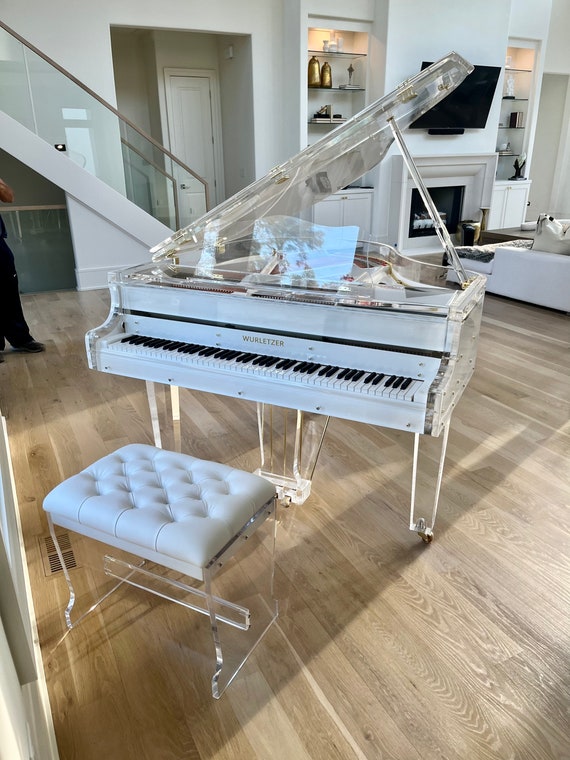This vertical, rectangular image captures the sleek, modern interior of a luxurious home. Dominating the center of the room is a stunning grand piano made entirely of clear material, giving it a translucent appearance. The piano keys remain traditional in design, while the rest of the piano—including its legs and raised cover—is completely see-through. In front of this striking instrument sits a matching clear bench, adorned with a tufted white cushion.

The room features light wood flooring that contrasts beautifully with the predominantly white and light gray walls. To the right side of the image, a blank black TV screen is mounted on the wall above an unused, white-outlined fireplace. Flanking the fireplace are built-in bookcases with what appear to be glass shelves, holding various decorative items. In the foreground, partially visible is a segment of a white couch, adding to the modern aesthetic of the space.

Behind the piano, a staircase with a clear plexiglass railing and a gray base ascends to what is likely the second floor. Adjacent to the staircase is a hallway leading to another room, marked by a white door. The overall composition and minimalist color palette emphasize the clean lines and contemporary feel of the home.